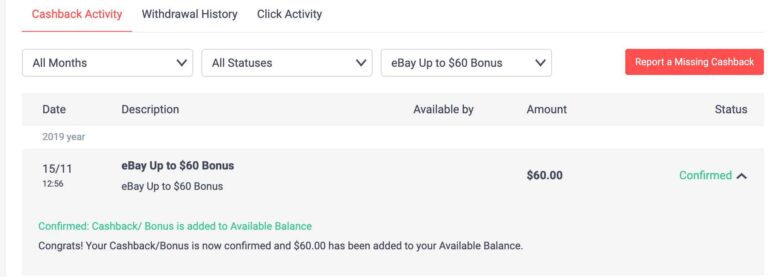A screenshot captures a digital dashboard, possibly from a financial tracking website or app. At the top of the interface, several elements are prominently displayed. The header features tabs and labels, including "Withdrawal History" and "Click Activity." There are also interactive drop-down menus labeled "All Months" and "All Statuses," along with a banner-like notification mentioning an "eBay up to $60 bonus."

Below these options, a structured table is visible, divided into multiple columns: "Date," "Description," "Available By," "Amount," and "Status." 

- The first row under "Date" shows the year "2019," but has no data in the subsequent columns.
- The second row under "Date," labeled "15/11," features "eBay up to $60 bonus" in the "Description" column, though other columns are not populated.
- The third row, marked "12:56," also lists "eBay up to $60 bonus" under "Description," with a corresponding amount of "$60" in the "Amount" column.

The "Status" column appears blank throughout. Additionally, "Cashback Activity" is highlighted in red at the top, possibly indicating a clickable or priority section. The visual layout suggests a focus on tracking specific transactions and potential bonuses, particularly related to eBay.